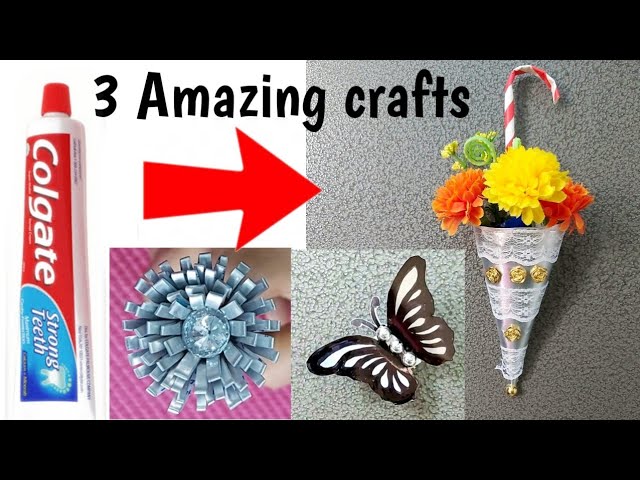The image titled "Three Amazing Crafts" features a visually striking collage against a varied background of white, gray, and purplish hues. At the top, bold black text announces the theme, with a prominent red arrow beneath it pointing from left to right. 

On the left, positioned on a white background, stands a vertically oriented tube of Colgate toothpaste, adorned with a red cap and text indicating it promotes strong teeth. The image of the toothpaste is bordered by a red arrow directing attention to the adjacent crafts.

Central to the display is an ornate cone resembling an ice cream cone but composed of shimmering gold, silver, and white materials. The intricate cone holds an arrangement of flowers and a candy cane, colored in vibrant hues of yellow, green, orange, and blue, suggestive of a festive bouquet.

On the lower level, within a purplish backdrop, lies a detailed chocolate butterfly, its black and white wings meticulously crafted around a diamond-like centerpiece. 

To the right, set against a gray and white background, is an exquisite floral object, resembling a paper flower with petals that fan out from a crystal-studded center. This display showcases the theme of innovative and artistic crafts, each piece offering a unique blend of materials and design.